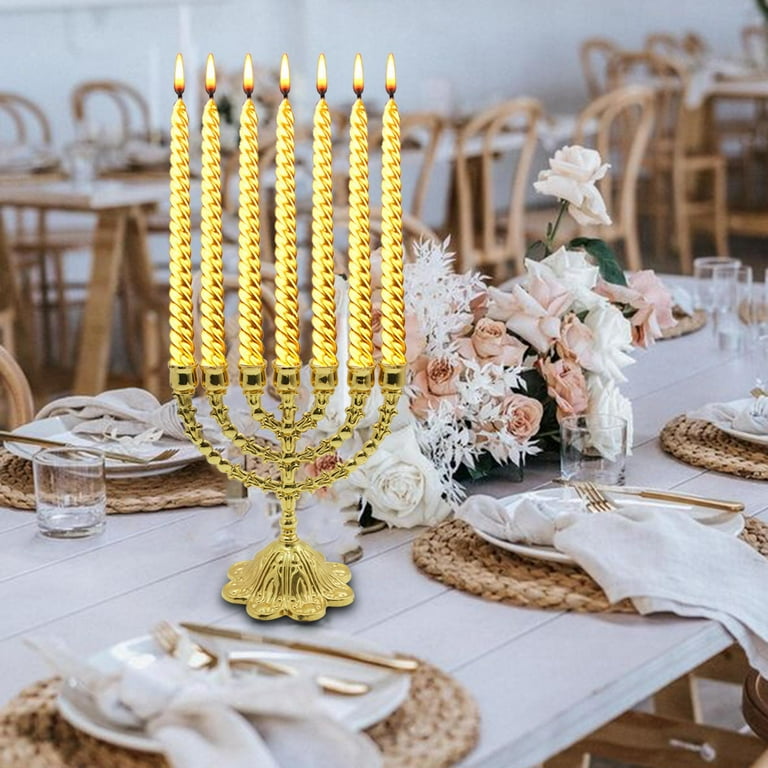The photograph features a beautifully set dining table with a prominent golden menorah at its center, holding seven spiral-braided candles with flames flickering atop them. The table is adorned with circular woven brown placemats, each topped with a small white saucer plate, a shiny gold knife and fork on one side, and a neatly knotted napkin on the other. An elegant floral arrangement of white and pink roses graces the middle of the table, adding a touch of freshness. Additional similarly set tables are visible in the background, enhancing the festive atmosphere.